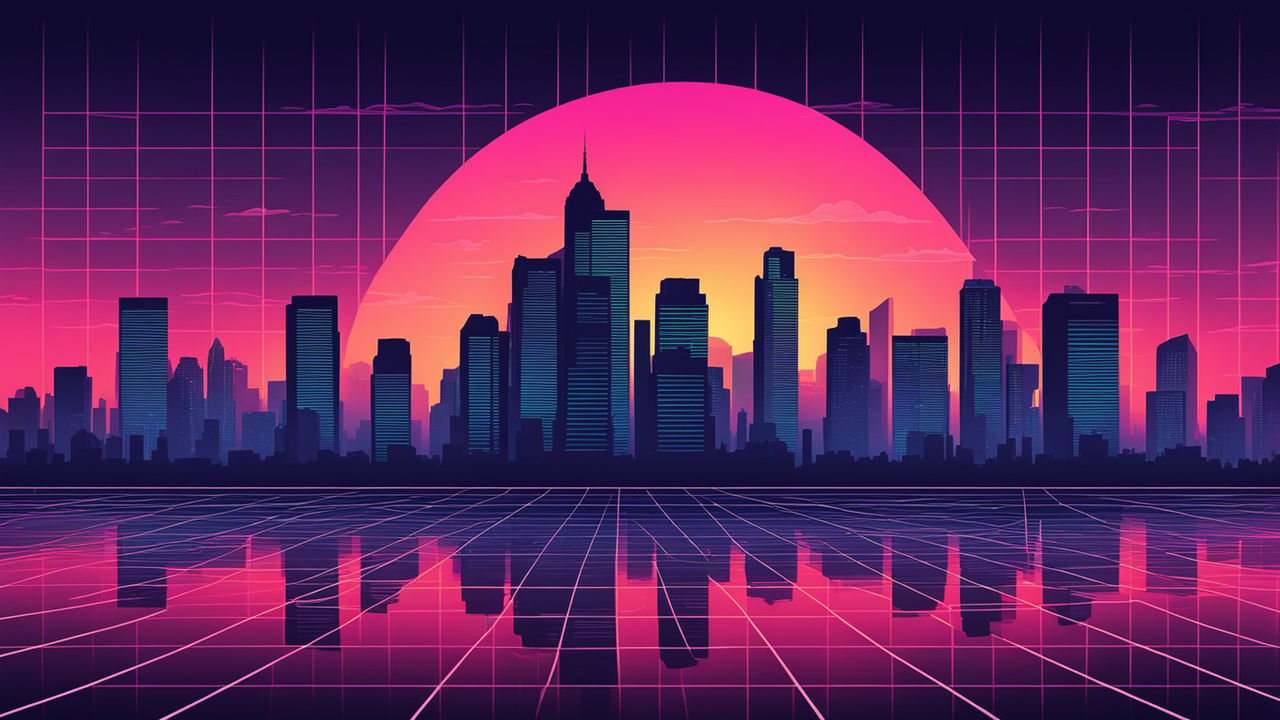This computer-generated illustration depicts a vibrant vaporwave-style cityscape that exudes classic 1980s aesthetics. Dominating the scene is a horizon filled with tall, spire-like skyscrapers, depicted in deep blue hues, climbing upwards. The backdrop features a massive sun rendered in a striking gradient that transitions from fluorescent pink and orange to a very strong yellow, suggesting either a rising or setting sun. Below this prominent sun, the sky transitions into a rich purple, intersected by a vivid pink grid pattern that extends towards the viewer, offering a sense of depth and dimensionality.

The lower half of the image mirrors the upper skyline, with the buildings' reflections cast upon a similarly styled grid that stretches out from the horizon, reinforcing the geometric precision typical of vaporwave art. Notably, while the sun itself is not reflected, its fluorescing pink and orange glow are. The grid lines behind the skyline and beneath it create a cohesive and striking visual experience. The edges of the composition fade into darker tones, adding a dramatic contrast that further highlights the luminous central elements. This detailed convergence of colors and geometric patterns captures the nostalgic essence of vaporwave imagery.